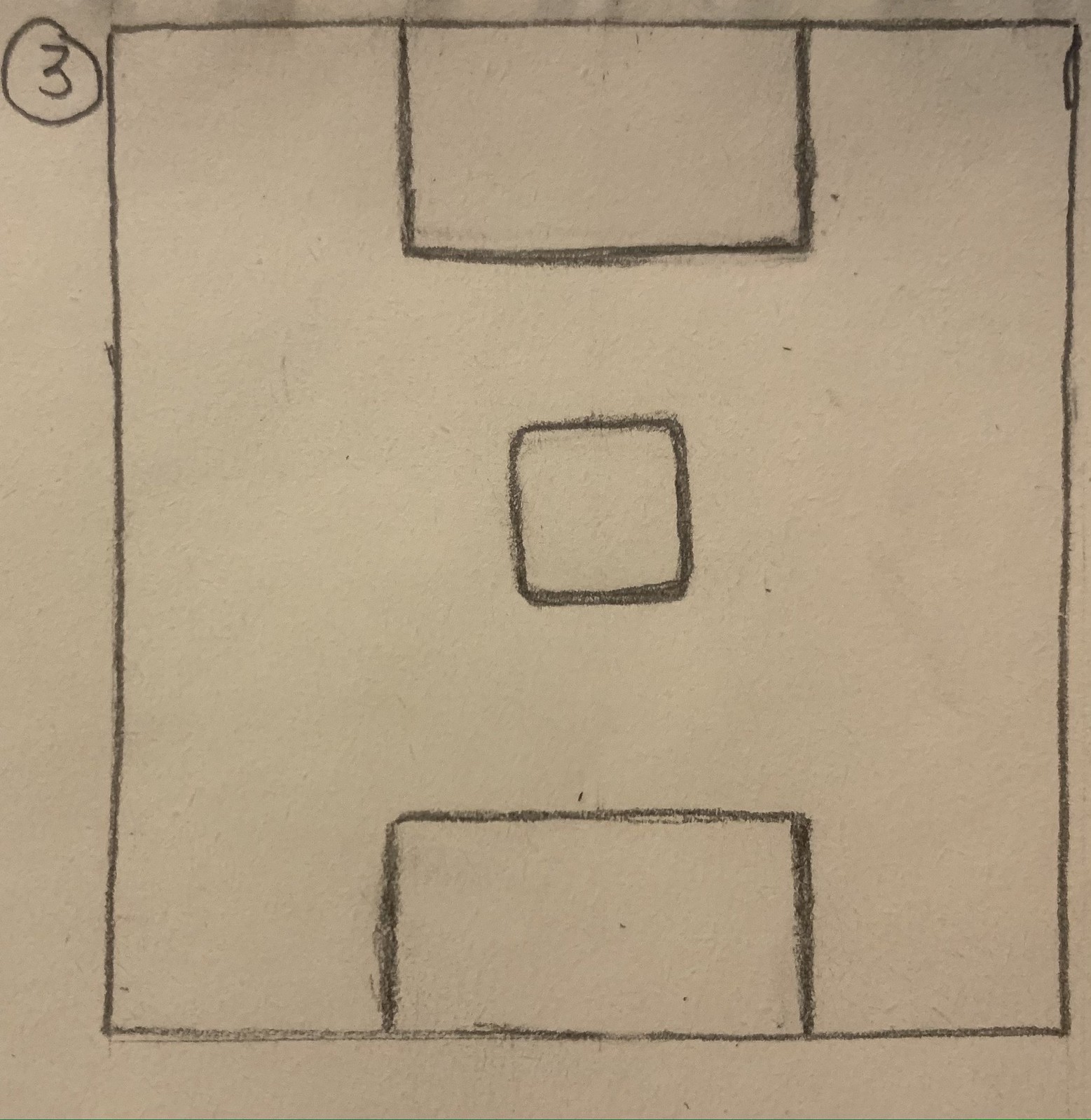This is a detailed photograph of a hand-drawn illustration, created using a black crayon or marker on an off-white sheet of paper. The overall image is square. In the upper left-hand corner, there is a black circle enclosing the number three. The central feature of the drawing is a large square outlined in black. Centrally placed on the top margin is a rectangle outlined in black, which exhibits slight smudging of the ink. At the very center of the illustration, there is a small black square. The bottom margin also features a black outlined rectangle. The composition of the image includes a large square with two rectangles—one at the top and another at the bottom—and a small square situated dead center between the two rectangles.